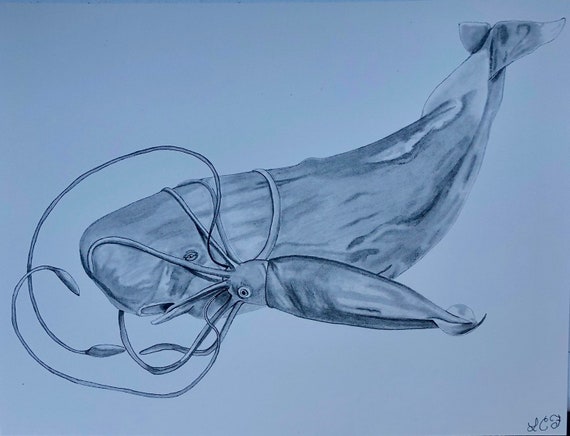This detailed and realistic pencil or charcoal-style drawing, created on light blue background paper, features a dramatic scene of a whale, possibly a sperm whale, locked in battle with a giant squid. The artwork, marked with the initials LC (or possibly LCJ) in the lower right corner, showcases intricate details such as striations and varying shades of grayish blues that highlight the texture and form of both creatures. The giant squid's tentacles are wrapped tightly around the whale's head, with one tentacle crossing its mouth and several ensnaring its body, conveying a sense of struggle and distress in the whale's expression. The monochrome palette enhances the intensity and realism of this evocative marine encounter.